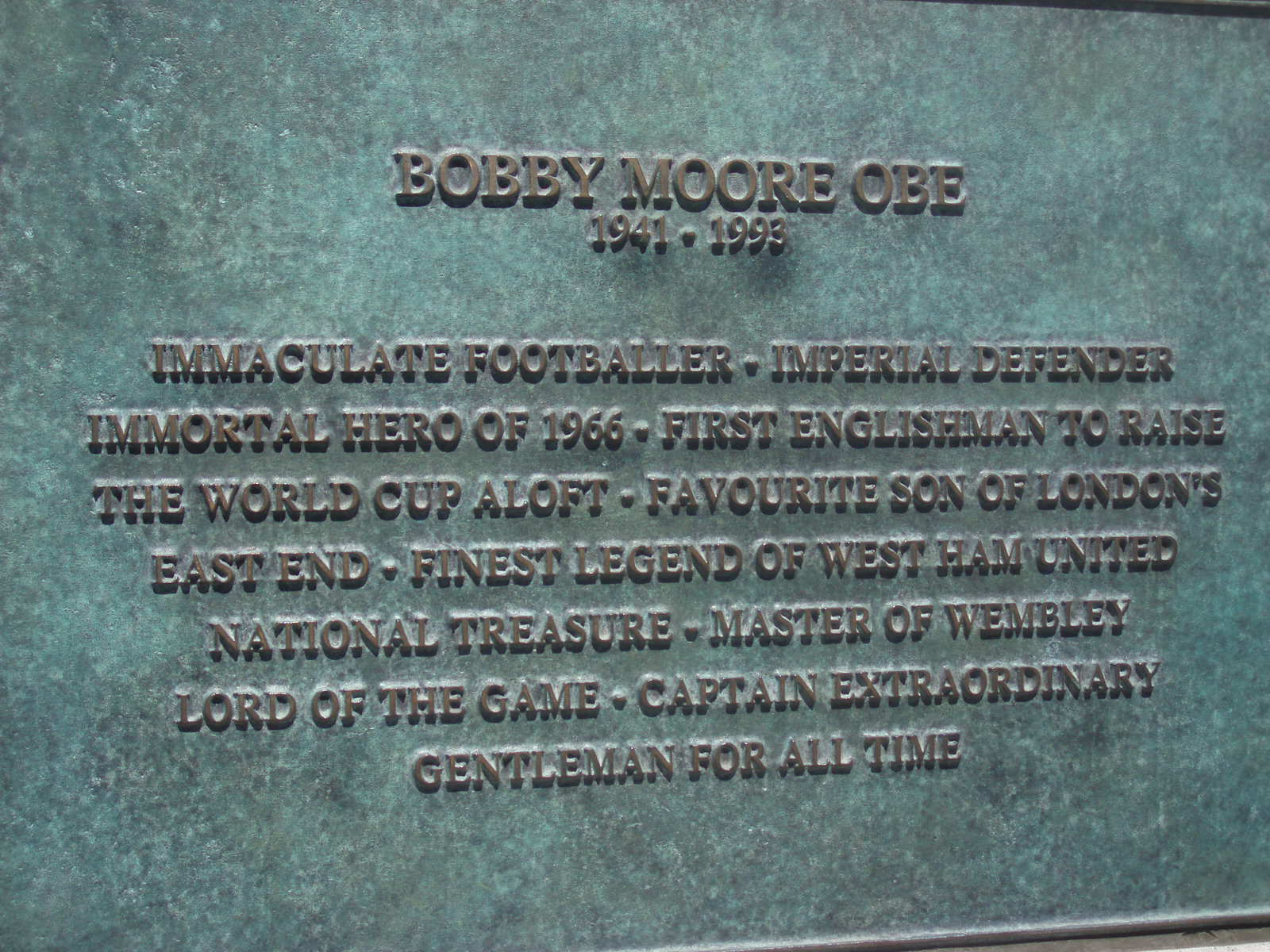This detailed and descriptive caption combines the key elements from each person's commentary:

This image depicts a close-up photograph of an outdoor memorial plaque, likely made of bronze, which has oxidized and turned green over time. The plaque is engraved with brownish-grey metal letters. It honors Bobby Moore, OBE, born in 1941 and deceased in 1993. The text on the plaque reads: "Bobby Moore, OBE, 1941-1993." Below his name, it celebrates his achievements and legacy with these inscriptions: "Immaculate Footballer, Imperial Defender, Immortal Hero of 1966, First Englishman to raise the World Cup aloft, favorite son of London's East End, finest legend of West Ham United, National Treasure, Master of Wembley, Lord of the Game, Captain Extraordinary, Gentleman for all time." Sunlight splashes on the plaque, but the larger context or structure it is mounted on is not visible in the photograph. The tribute exudes respect and admiration, highlighting Bobby Moore's esteemed position in football history.